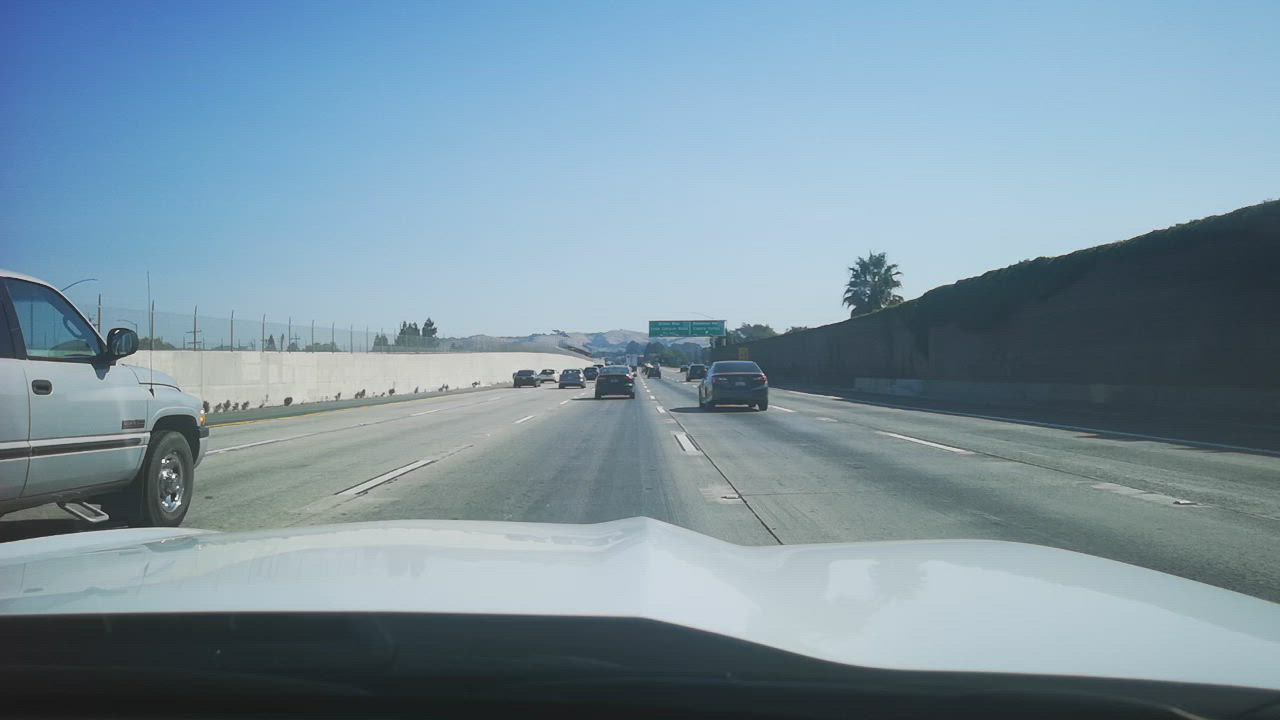This image, likely captured from inside a car using a dash cam or cell phone, depicts a busy five-lane highway. The perspective from within the car hints that it may be a white, light gray, or silver vehicle. Dominating the left lane, closest to the car, is a smaller truck, possibly an S10, in a similar color scheme of white, light gray, or silver. Spanning the highway, a notable number of vehicles populate the lanes, many in dark hues such as shades of dark blue, dark gray, and black. Background elements include an array of palm trees and regular trees lining the highway, contributing to a scenic atmosphere. A prominent green highway sign, segmented into three parts, provides navigational information. Separating the lanes of opposing traffic is a medium-height gray concrete barrier, adding to the structured layout of this vibrant roadway scene.